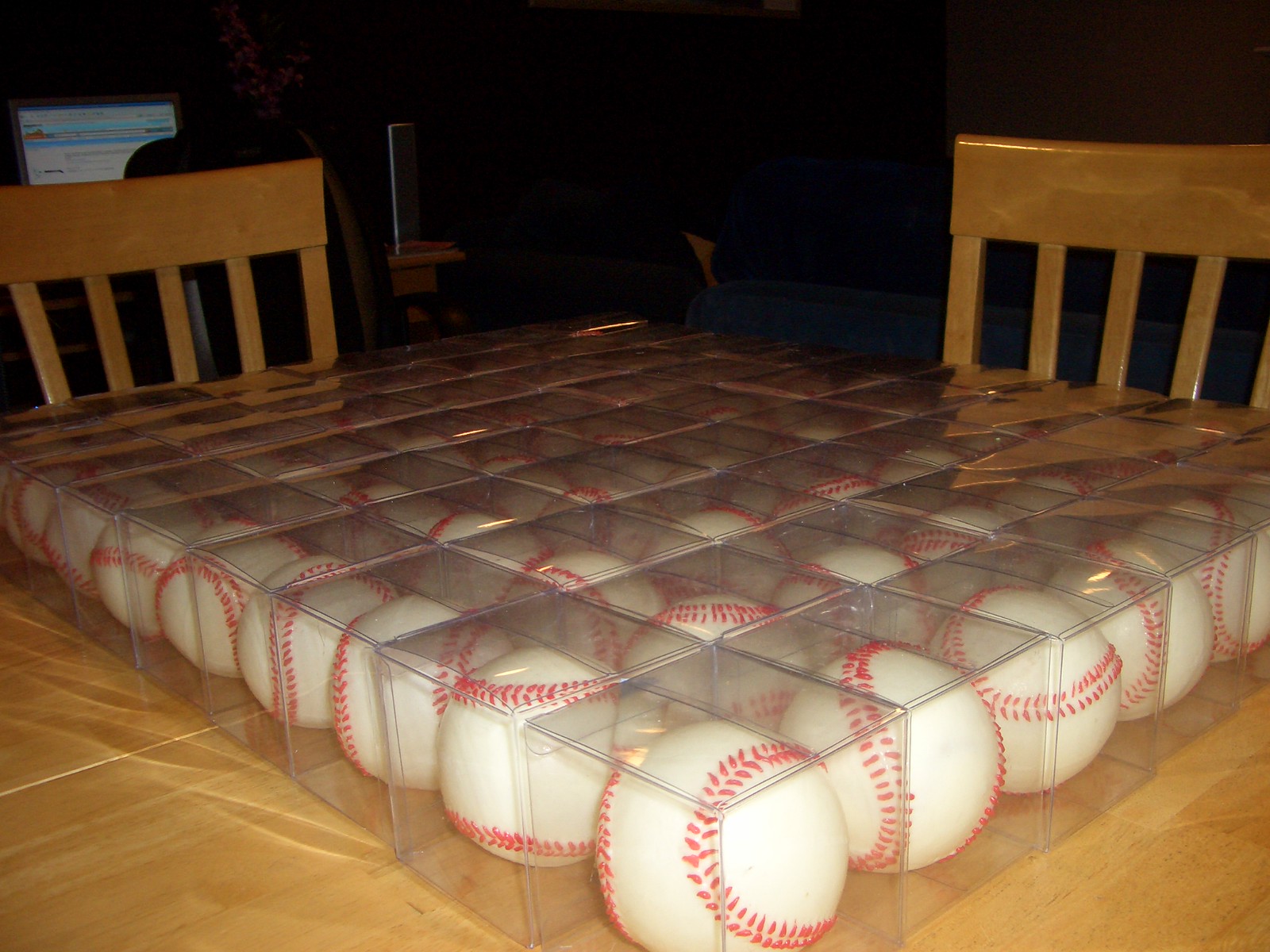The photograph captures a wooden dining table nearly entirely covered with transparent, cube-shaped plastic cases, each holding a single baseball. The baseballs are arranged in a precise, highly satisfying formation comprising seven rows and nine columns, totaling approximately 63 baseballs. The balls are new, displaying their white surfaces and bright orange stitching. The table, made of yellowish wood, is accompanied by two matching wooden chairs positioned at the back. In the dimly lit background, the glow of a computer screen is visible on the left side, partially illuminating the shadow of a desk chair in front of it.